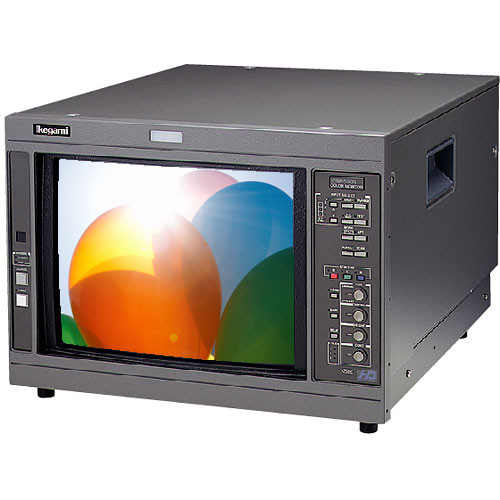The image depicts a full-color photograph of a box-like electronic device with a handle, indicating its portability. The box is gray with four black rubber feet on the bottom. It is set against a white background. Prominently featured is a screen on the front that displays multicolored balloons in hues of orange, green, blue, and purple, with a bright light, possibly the sun, emanating from the top. To the right of the screen, there is a detailed control panel, featuring numerous silver knobs and buttons arranged vertically, including four distinct knobs and 13 buttons. On the left side, there are two additional buttons. The screen and control panel are joined by a thinner border on the left side. Though slightly blurry, there is a label or name on the device that appears to say "Kermy."